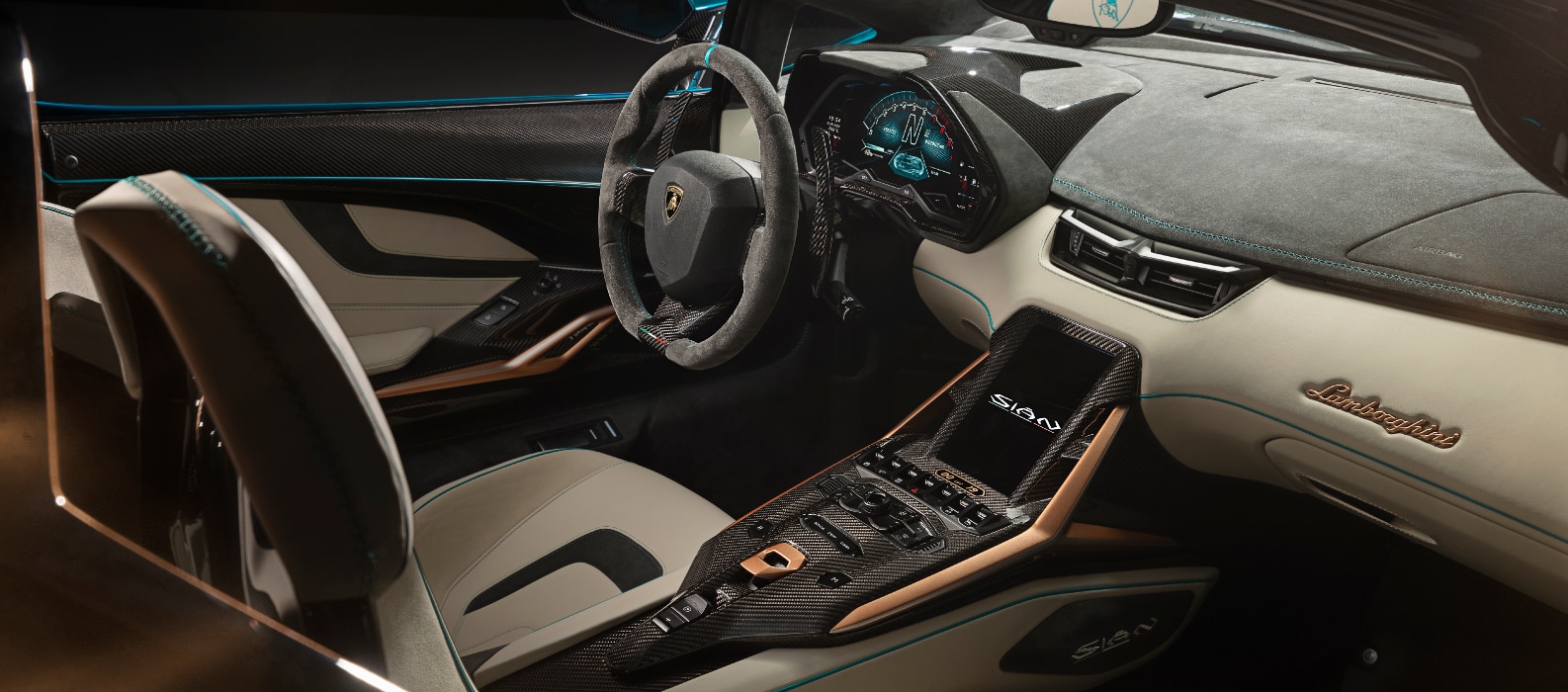This image captures the refined interior of a Lamborghini, emphasized by luxurious materials and an elegant design. The focal point is the black Alcantara-wrapped steering wheel featuring the Lamborghini logo. Surrounding this is a meticulously crafted light gray dashboard adorned with high-quality Alcantara fabric. The dashboard includes a digital display showing an "N" for neutral and a speedometer with a blue hue.

Central to the interior is the carbon fiber center console, detailed with numerous buttons and a screen with white text (though its specific content is unreadable). The console features a mix of black and orange tones, adding to the modern aesthetic.

The seats, upholstered in a combination of beige leather and black stripes, exude comfort and sophistication. The Lamborghini script in cursive can be seen above the glove compartment on the passenger side, while the center console features a subtle "Sian" label.

The car's craftsmanship is evident in every detail, from the beige leather lower dashboard to the golden Lamborghini stitching. The doors continue the color theme with blue, white, and black accents. The overall interior is a harmonious blend of black, beige, and light gray, set in a horizontal landscape orientation that captures the luxurious spirit of this high-end sports car.